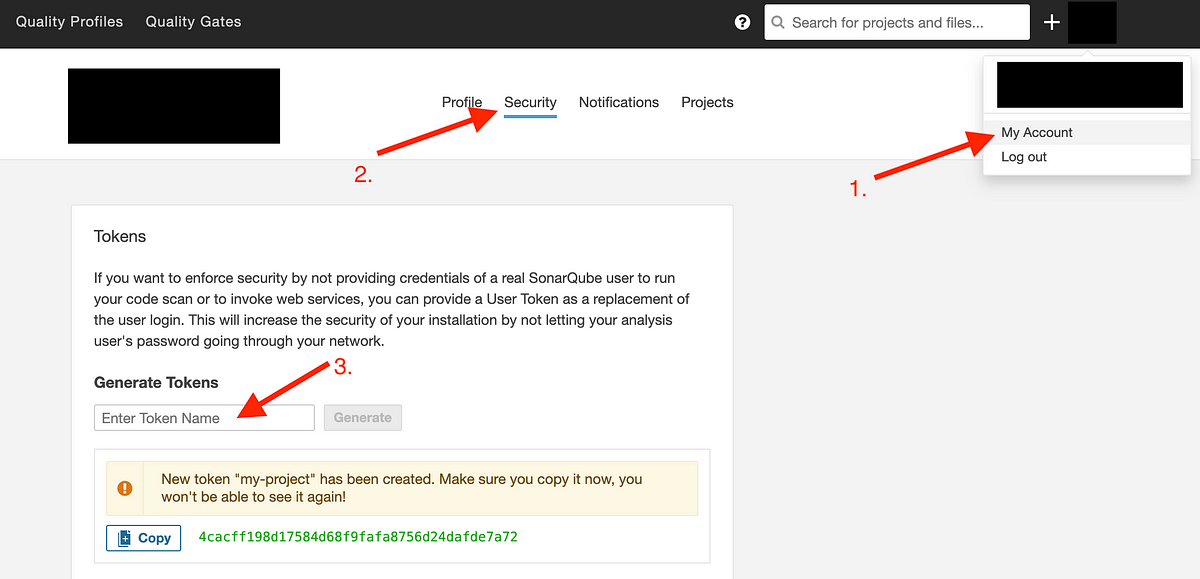Screenshot Description:
This screenshot captures a section of a software management interface, specifically focusing on user security settings.

At the top of the image, there is a black border. On the left side of this border, the text "Quality Profiles" is displayed, followed by "Quality Gates" slightly to the right. Towards the far right side of the border, a search bar is visible, accompanied by a plus sign to its right.

The main part of the screenshot features a white background. In the top left corner, there is a small black rectangle. Centrally located on the screen is a white box displaying various tabs: "Profile," "Security," "Notifications," and "Projects." The "Security" tab is underlined in blue, indicating it is the active selection.

On the far right of the screen, another black rectangle is visible featuring a drop-down menu with options for "My Account" and "Log out." A red arrow labeled with the number "1" points towards "My Account."

In the central area of the screen where the "Security" tab is selected, another red arrow labeled "2" points towards this tab. Directly beneath this, a white rectangle labeled "Tokens" explains the purpose of user tokens: "If you want to enforce security by not providing credentials of a real SonarQube user to run your code scan or to invoke web services, you can provide a user token as a replacement of the user login. This will increase the security of your installation by not letting your analysis users' passwords go through your network."

Further down, the option to "Generate Tokens" is displayed, along with a bar to enter a token name. A third red arrow, labeled "3," points towards this input field.

At the very bottom of the screen, there is a yellow bar containing the message: "New token. My project has been created. Make sure you copy it now. You won't be able to see it again." Below this message, a generated code is shown alongside a "Copy" button.